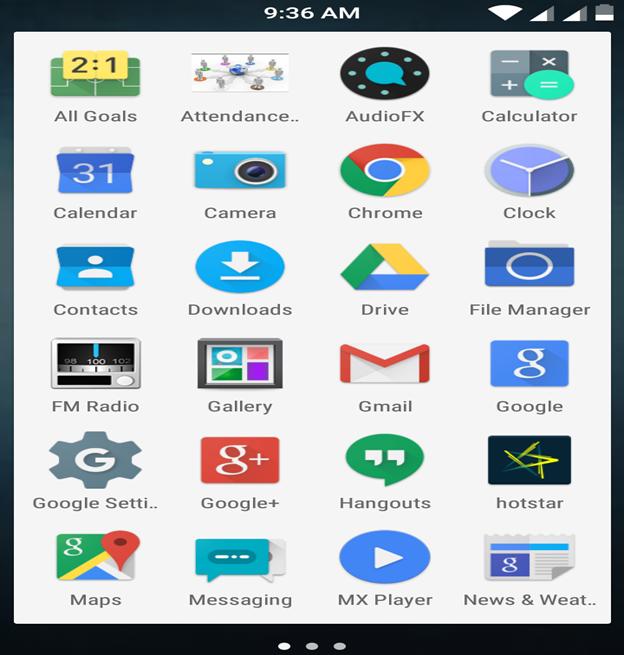The image showcases a cell phone screen displaying the app menu. The screen is bordered by a dark black or navy blue header, footer, and thin edges. At the top of the screen, "9:36 AM" is prominently displayed in white text. Adjacent to the time, on the top right corner, are icons indicating Wi-Fi connectivity, signal strength, and battery status. 

Centrally located at the bottom of the image are three small gray dots, suggesting multiple pages of apps. Dominating the majority of the image is a large vertical white rectangle containing the apps. The apps are organized into six rows and four columns, each accompanied by a colorful icon and labeled beneath.

From left to right and top to bottom, the apps listed are:
1. All Goals
2. Attendance
3. Audio FX
4. Calculator
5. Calendar
6. Camera
7. Chrome
8. Clock
9. Contacts
10. Downloads
11. Drive (Google Drive)
12. File Manager
13. FM Radio
14. Gallery
15. Gmail
16. Google
17. Google Settings
18. Google Plus
19. Hangouts
20. Hotstar
21. Maps
22. Messaging
23. MX Player
24. News and Weather

Each piece of text is appropriately positioned below its respective icon, providing a clear and organized view of the user's app selection.